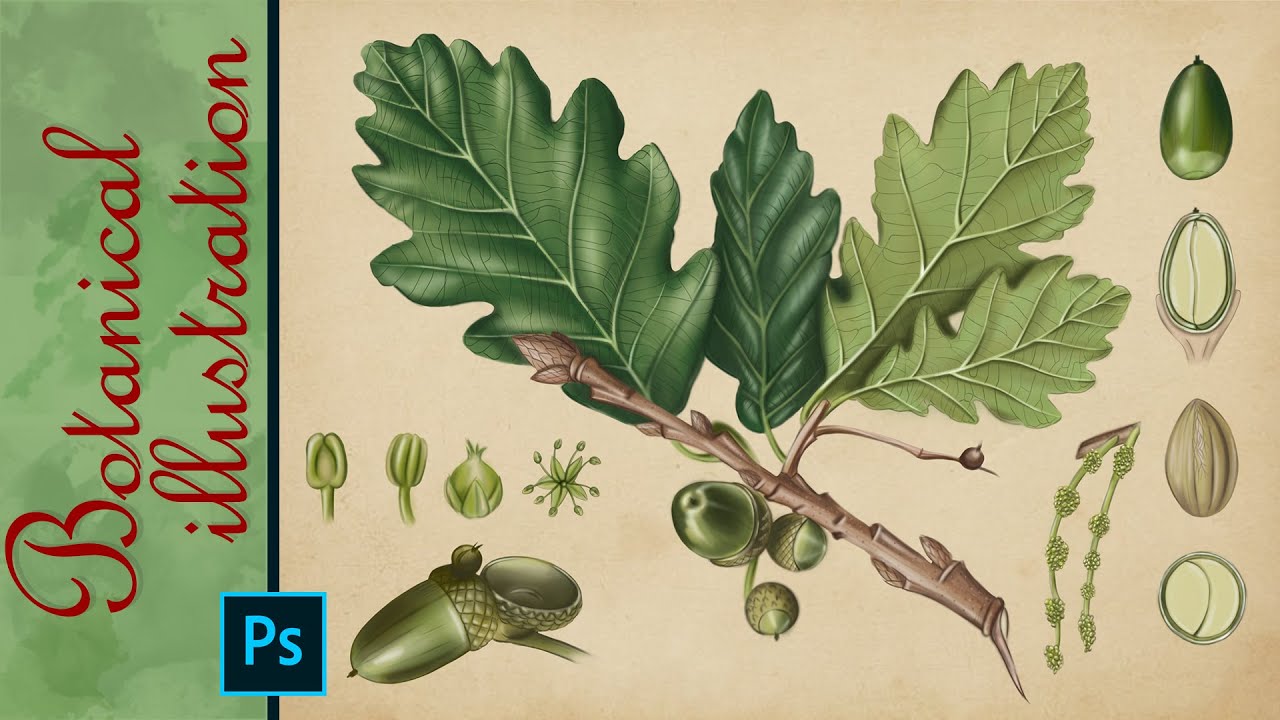The image appears to be the front cover of a book laid sideways. The title "Botanical Illustration" is written in red cursive on a vertical green border located on the left-hand side. Below this, there is a blue square with the letters "PS" in blue as well. The main body of the cover is an off-white or cream color, featuring an intricate illustration of an oak branch. The branch, depicted in brown, supports several clusters of green leaves, each varying slightly in shade and featuring rounded edges with pointed tips.

To the right of the branch, there are detailed drawings of acorns and seeds in different stages. At the top, there's a green acorn, followed by an illustration of it cut in half to reveal its interior. Below this is a brown seed and then another more circular seed with a green line across it. Scattered around the page are smaller drawings illustrating the flower blooms that eventually develop into acorns, providing a botanical breakdown of the fruit's growth and structure.